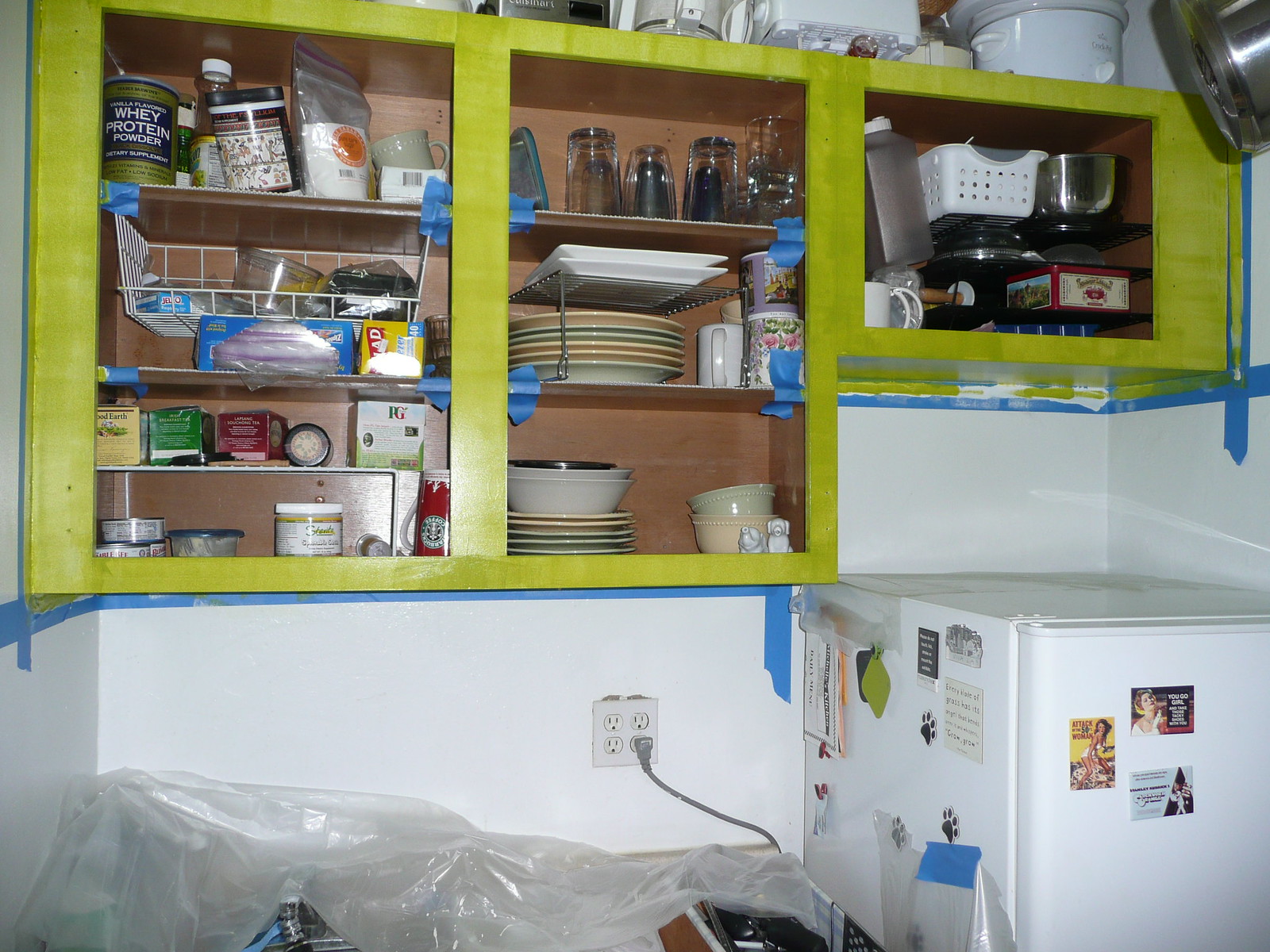The photo captures a kitchen scene in the midst of a renovation. The open cupboards reveal an assortment of items, including plates, mugs, glasses, tea cartons, whey protein powder, and other miscellaneous goods. Painter's tape and masking tape can be seen around the edges, hinting at recent painting activity. A plastic cover is draped below, likely to protect surfaces from paint splatters. The cupboards are currently painted a not-so-appealing shade of yellow, which might still be awaiting a final coat.

Above the cupboards, various kitchen appliances such as a slow cooker, blender, and toaster are visible. On the right side of the image, a refrigerator, plugged into an American-style outlet, is adorned with a few magnets. Notably, one magnet appears to be a movie poster for "Attack of the 50 Foot Woman," while others feature different women. The white walls of the kitchen also contain outlets, and a stove, partially covered with plastic, sits below the workspace.